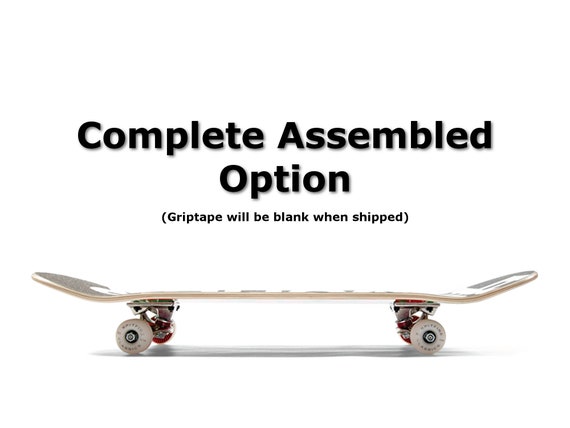This image appears to be from an online shopping website or a catalog, depicting a skateboard on a plain white background and surface aimed at potential buyers. The skateboard is presented in a side view, showcasing the white wheels with red trim on the inside. Above the skateboard, in bold black text, it reads "Complete Assembled Option," with a note in parentheses below stating "Grip tape will be blank when shipped." The grip tape on top of the skateboard, though not fully visible, seems to have a black color with an indistinct white design. The ends of the skateboard deck are slightly elevated, and a faint shadow can be seen beneath it. This detailed display aims to inform customers that the skateboard will arrive fully assembled, though without any pre-applied designs on the grip tape.